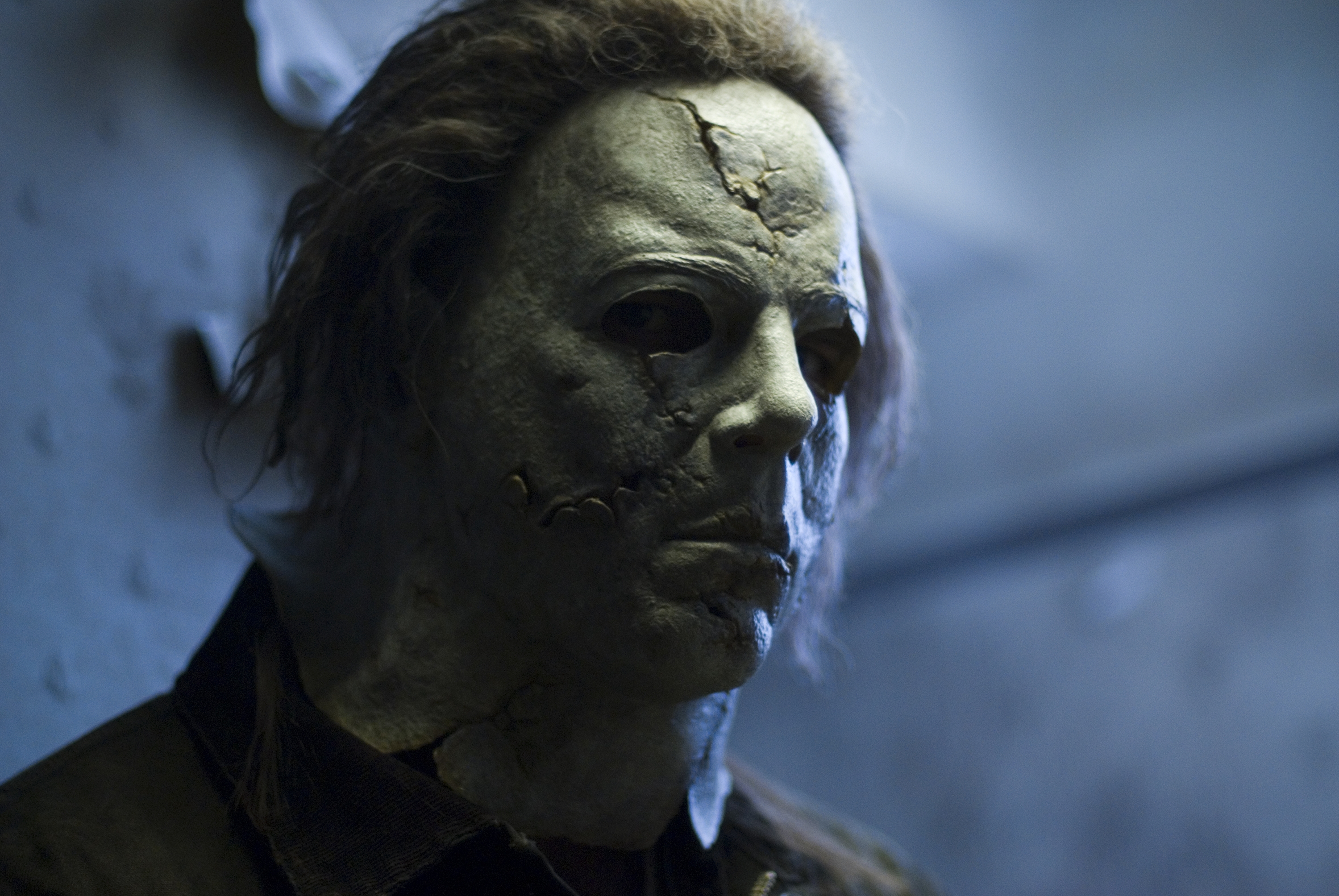The image presents a close-up shot of a man wearing a cracked, flayed mask resembling a disfigured face with noticeable scars. The mask emphasizes a somber, serious expression, with the real eyes being the only visible flesh through the mask's eye holes, adding a sense of mystery and menace. He has long, flowing brown hair that extends from underneath the mask, contrasting starkly with the mask’s white, aged appearance. The setting appears to be indoors with a blurred background, hinting at a grayish-blue wallpaper featuring floral patterns on one side. The individual is dressed in a high-collared shirt, partially visible from the top portion of the torso, enhancing the character's eerie, horror movie aesthetic reminiscent of Michael Myers from Halloween.